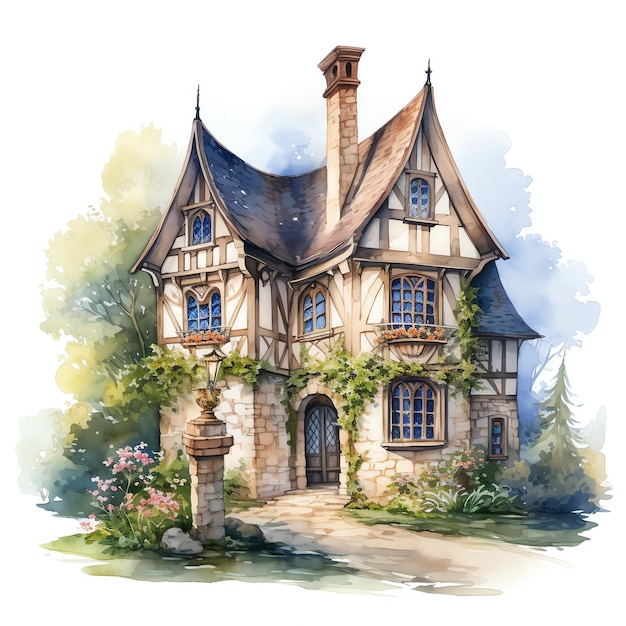This image depicts a picturesque painting of a large, old-fashioned cottage, reminiscent of the English countryside. The three-story house features multiple windows, seven in total, with lead glass paneling, and arched doorways. The house is primarily brown and white with a concrete lower level, topped by a brown, pointed roof with three peaks and a chimney. Additionally, two decorative spires and a smaller roof can be seen in the background. Ivy climbs up to the second story, adding charm to the structure. Surrounding the cottage are lush trees—some green and some with a bluish hue—and a notable pine tree in the front. The scene is dotted with vibrant flora, including pink flowers on the left side of the house and more in the foreground. A cobblestone walkway leads to the gray barred entrance door, and a brick light post with stone surroundings and flowers stands to one side, completing the idyllic setting. The artwork, likely a watercolor given its soft, muted palette of beiges, browns, blues, greens, and touches of pink, beautifully captures the serene atmosphere of this quaint homestead.